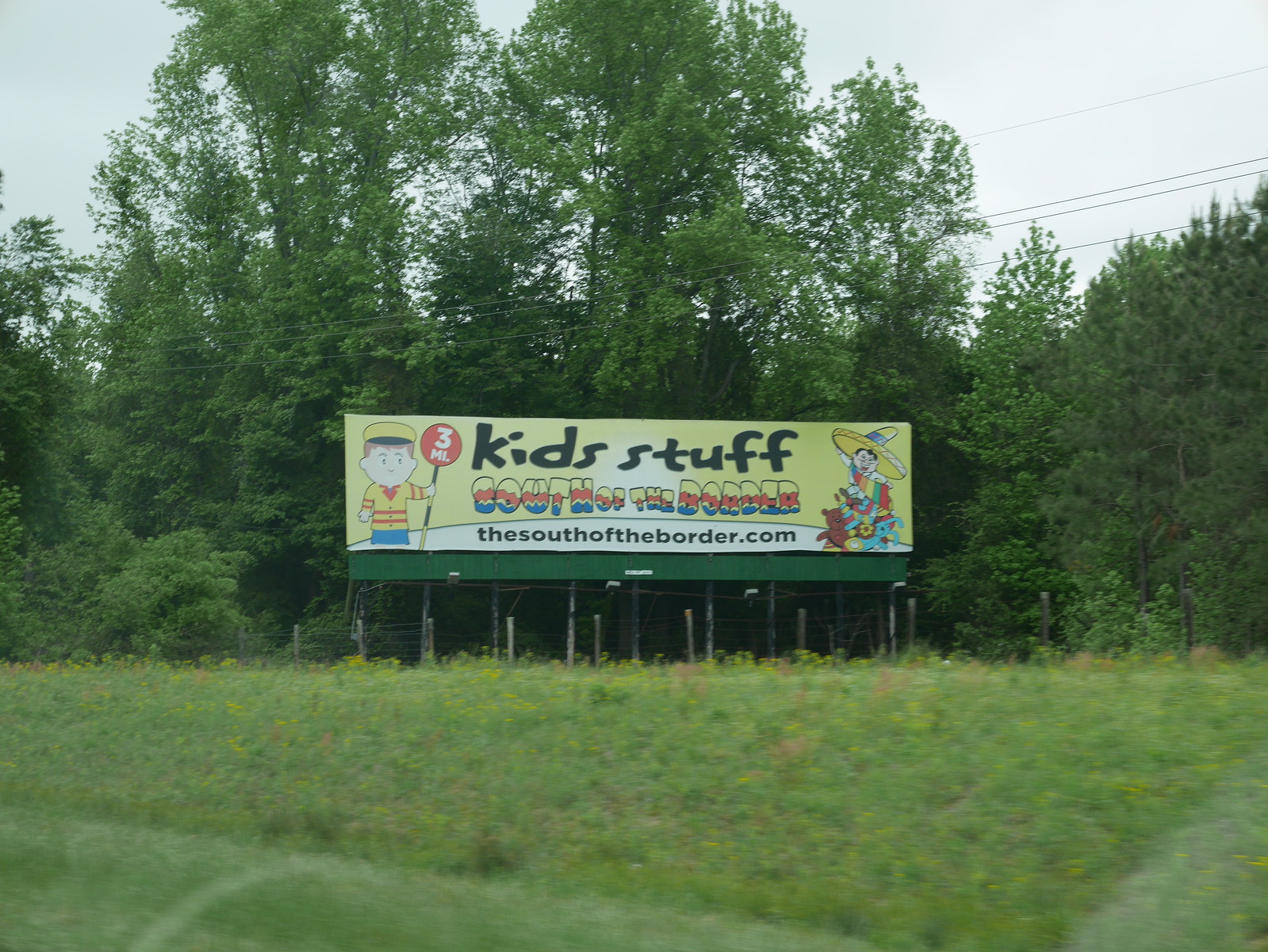In this photograph, an overgrown field of towering weeds and grass stretches out, giving the impression that it hasn't been mowed in a very long time. Bordering the field is a dense backdrop of various trees, including what appear to be taller trees at the center and pine trees on the right. Strung across the image, from left to right, are several power cords. Dominating the scene is a large billboard advertising "Kid Stuff South of the Border," accompanied by the website address, "TheSouthoftheBorder.com." The billboard features a colorful and vibrant illustration of a Mexican man dressed in a sombrero and a colorful scarf, with various toys on his lap. To the left of the man, an additional figure of a police officer clad in a yellow sweater with red stripes and blue pants holds a sign indicating "3 miles."